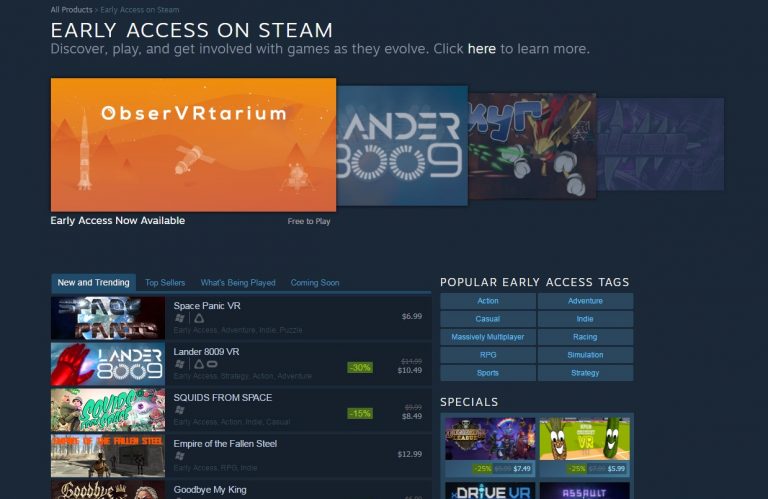The image showcases a Steam application interface highlighting early access games. At the top, a header reads “All Products Early Access on Steam” in bold white text. Beneath, a promotional message encourages users to "Discover, play, and get involved with games as they evolve. Click here to learn more."

Displayed prominently is the “Observer Trailer” with a vibrant orange background featuring space-themed effects and satellite imagery. Accompanying text reads “Early Access Now Available. Click to Play.” Adjacent to this, the game “Ender 3.0.0.9” is partially visible, with other game previews extending off the screen to the right.

Lower on the page, the section titled “New and Trending” lists several games:
- "Space Panic VR" priced at $6.99.
- "Lander 8.0.0.9 VR" available at a discounted rate of $10.49 (30% off).
- "Quits from Space" offered for $8.49 (15% off).
- "Empire of the Fallen Steel" priced at $12.99.

To the right, under the “Popular Early Access” banner with a dark blue background, game genres are listed in blue text, including Action, Adventure, Casual, Indie, Massively Multiplayer, Racing, RPG, Simulation, Sports, and Strategy.

At the bottom right, a “Specials” section indicates that there are games with a 25% discount, though specific game names are not provided. This well-organized display provides a comprehensive look at what’s new and trending in early access on Steam.